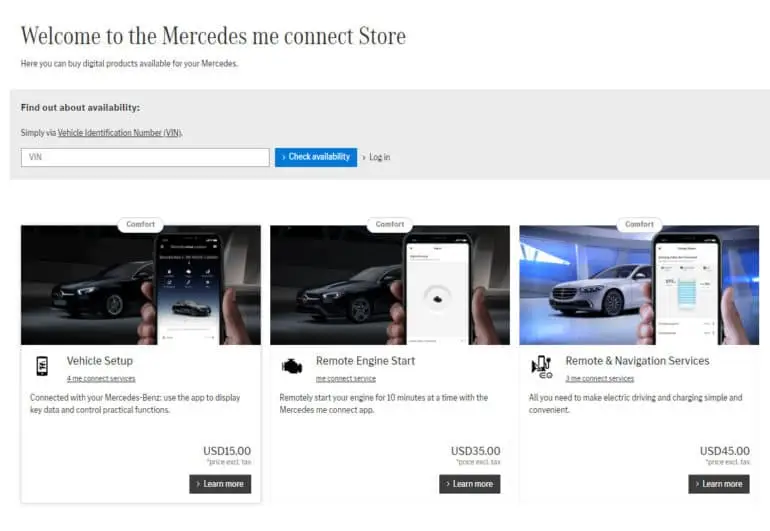Caption:

The Mercedes me connect store webpage is designed with a clean, white background and sleek black text at the top, welcoming visitors to explore digital products for their Mercedes. A prominent light gray rectangle beneath the header features the message "Find out about availability simply via vehicle identification number," followed by a white search bar labeled "VIN" and a blue button with "Check Availability." Next to it, there's a "Log In" option.

Below this section, three informational squares are displayed side-by-side:

1. The first square showcases a black sedan with a white "Comfort" bubble at the top center. On the right, a man's hand holds a smartphone displaying car details. The text beneath explains that you can use the app for vehicle setup and to view key data and control various functions. This service is priced at $15, with a "Learn More" button in a black rectangle.

2. The middle square features the same image but with a white background and a circle on the smartphone screen, highlighting the "Remote Engine Start" capability. This allows you to start your engine for up to 10 minutes using the Mercedes me connect app, priced at $35, and includes a "Learn More" button.

3. The third square presents a white sedan and a hand holding a phone that displays remote navigation services. The accompanying text describes how these services simplify electric driving and charging. This feature is offered at $45, with an option to "Learn More" in a black rectangle at the bottom.

Each of these sections provides users with detailed information on specific digital products available for enhancing their Mercedes-Benz experience.